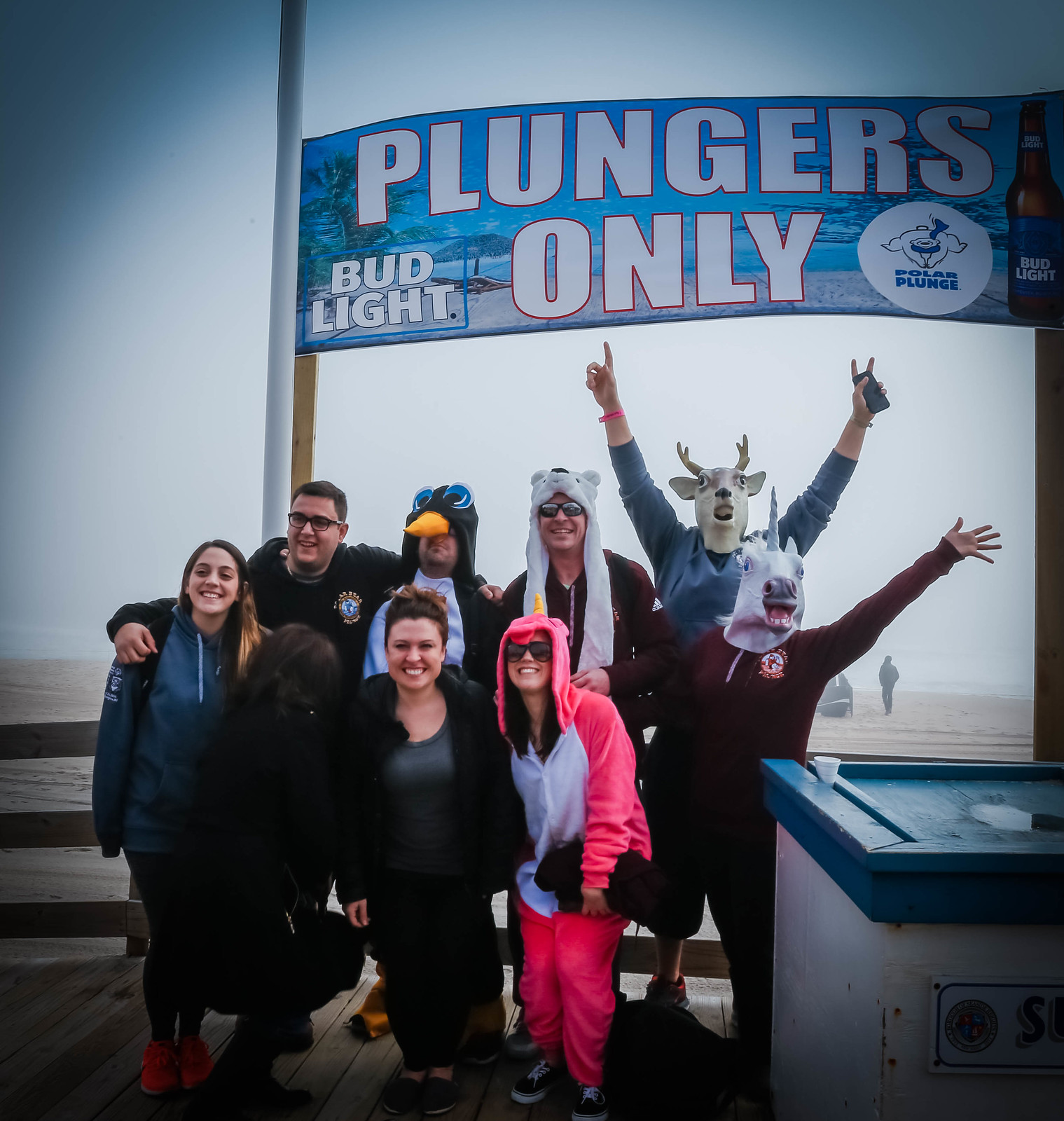The photograph captures a lively group of 10 people standing together at the beach, likely participating in a Polar Plunge event early in the morning. Dominating the top of the scene is a large banner with the words “Bud Light,” “Plungers Only,” and “Polar Plunge,” alongside an image of a Bud Light bottle. The backdrop clearly reveals the beach, complete with sand and a glistening ocean, and a few other individuals heading towards the water. Adding an element of fun and whimsy to the photo, several participants are dressed in festive costumes: someone in the back is dressed as a penguin, while another person up front sports a unicorn outfit. Additionally, there are masks and hats resembling a panda bear, a moose, and another unicorn. Five of the group members are visibly smiling, contributing to the cheerful spirit of the event. To the right side of the group, a booth is partially visible, possibly part of the event setup.